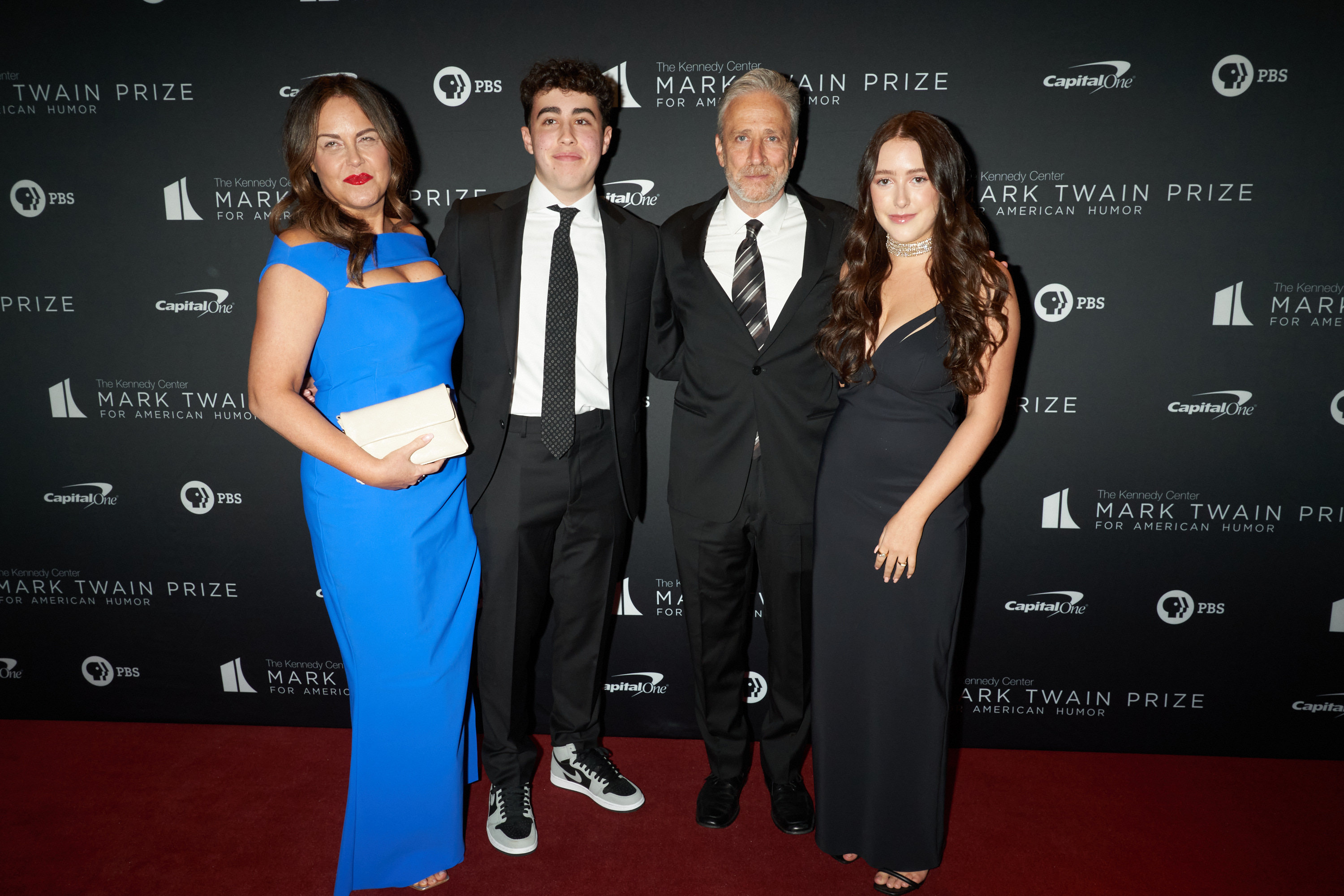In this image, we see four individuals posing directly at the camera, standing on a reddish carpet. The backdrop features a black banner with white text, indicating the event as the "Mark Twain Prize for American Humor," and includes advertisers such as Capital One and PBS. From left to right, the group consists of: a young woman with long dark hair, wearing a long black dress and sandals; a man in a gray suit with gray hair, a white shirt, a striped black and white tie, and shiny black shoes; a younger man with dark hair in a black suit, white shirt, black tie, and tennis shoes; and an older woman with dark hair in a long blue dress, holding a small white purse. The setting appears to be indoors at an event, with the image capturing a mix of colors including black, white, gray, blue, red, and brown.